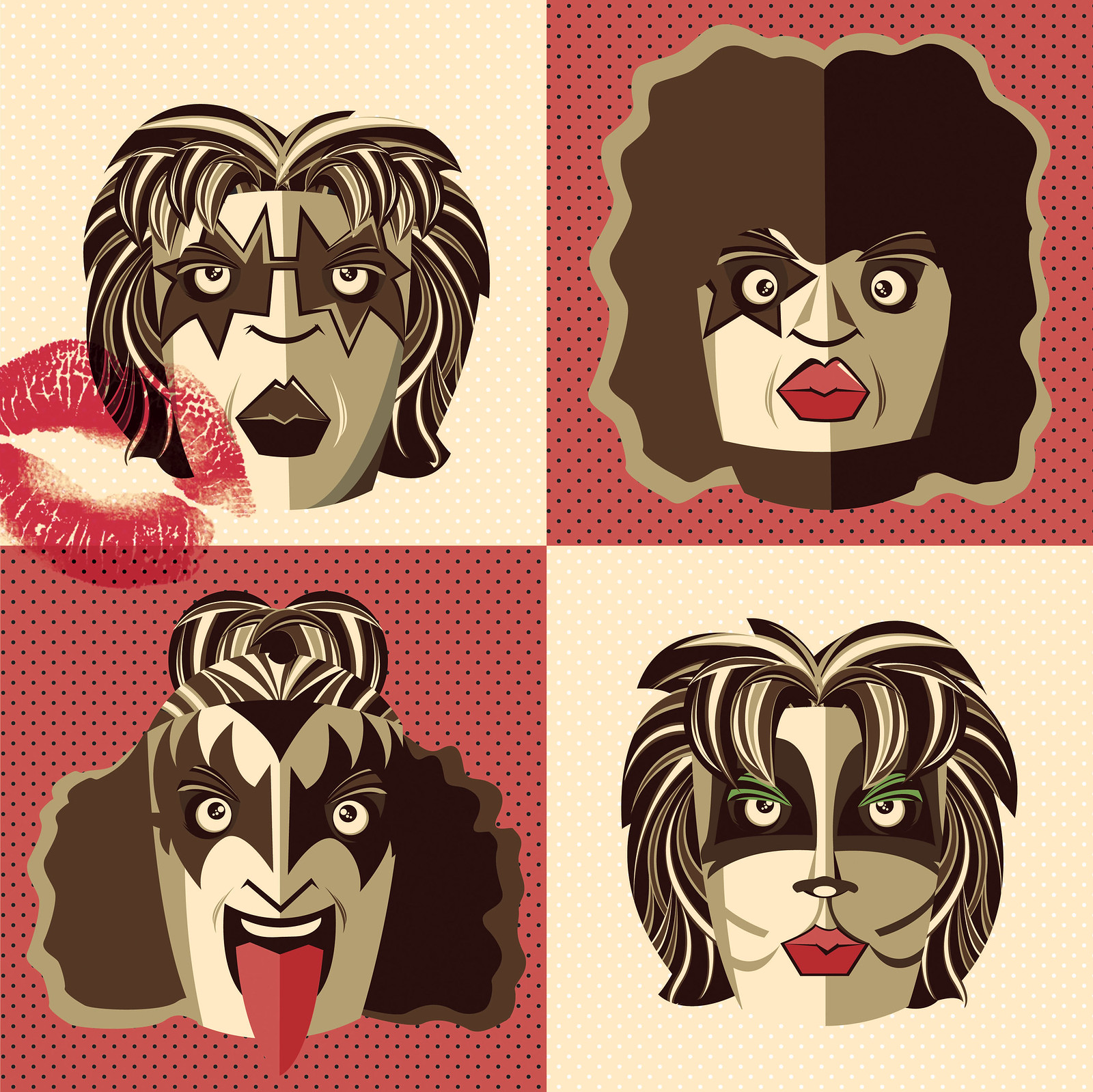This image is a computer-generated, cartoon-styled interpretation of the band KISS, presented in a multi-panel layout. Each panel distinctly portrays a member of KISS with their signature makeup and hairstyles.

The top left panel features a man with short wavy hair and a dark star pattern around his eyes. His lips are thick and black, against a cream background with white dots. A bright red lipstick kiss mark overlays this panel, seemingly migrating towards the bottom left.

In the top right panel, a man is shown with wavy black hair and a black star pattern over his left eye. He sports thick red lips, set against a red background with black dots.

The bottom left panel displays a depiction of Gene Simmons, identifiable by his bushy hair, partially pulled up, and his infamous extended tongue. His eyes are accentuated with dark makeup. This image features a red background with black dots.

The bottom right panel shows a man with cat-like makeup, including a blacked-out eye area, cat nose, and whiskers. His hair is a mix of layered black, white, and grey strands, matching the cream background with white dots.

This pop art-esque, graphic design captures the essence of KISS with a blend of white, cream, red, and black tones, underscored by striking accents such as the red lips and vivid lipstick kiss mark.